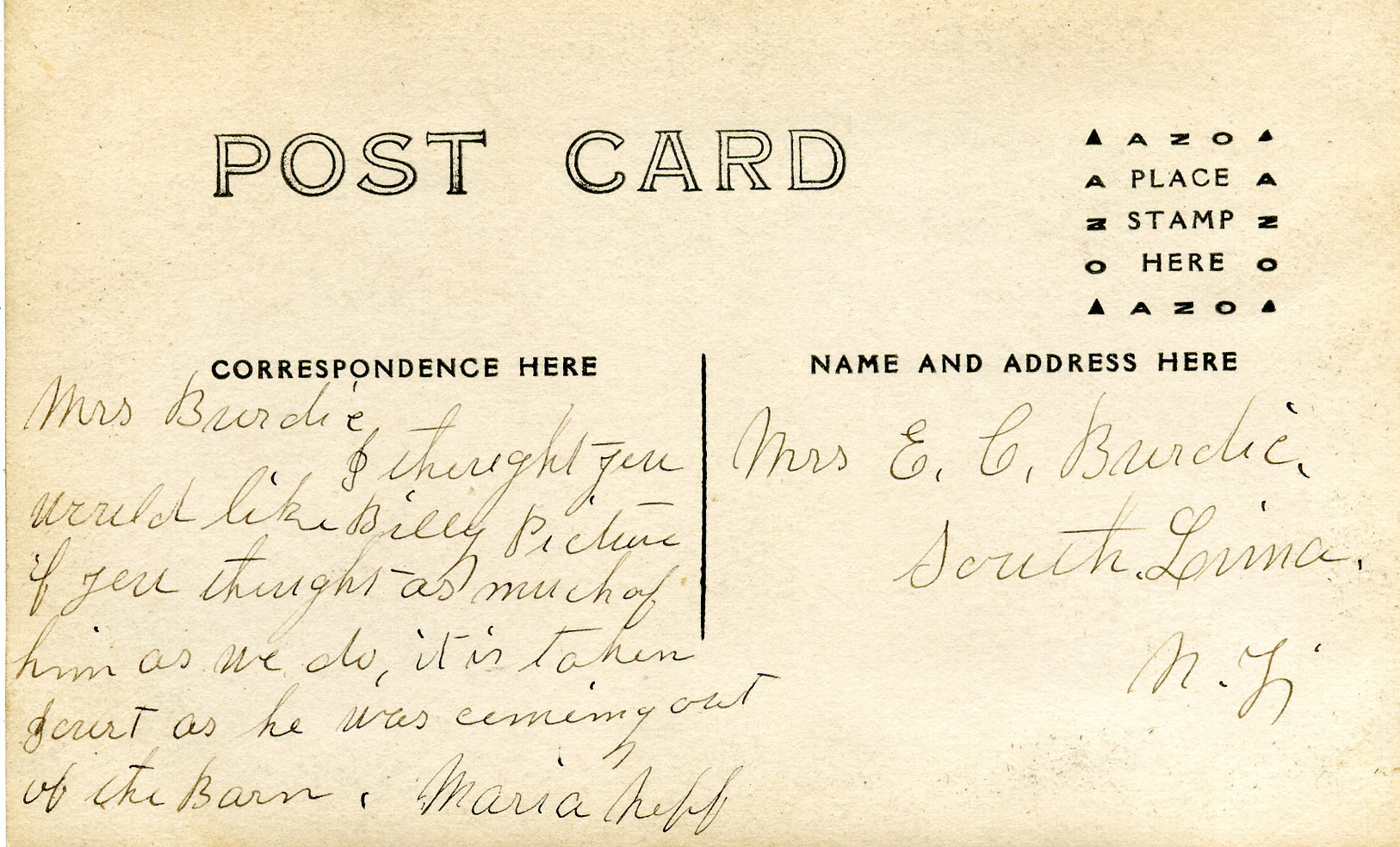The image depicts the back of an aged, off-white or cream-colored postcard, which is divided into two sections by a thin vertical line. At the top, the word "POSTCARD" is written in bold, black outlined capital letters. On the left section, under the header "CORRESPONDENCE HERE" in bold, there is a handwritten note: "Mrs. Brody, I thought you would like Billy's picture if you thought as much of him as I do. It has taken something as he’s coming out of the barn. Maria Muff." The handwriting is in a cursive script. To the right of this section, across the vertical divider, is a designated area for the recipient's information with "NAME AND ADDRESS HERE" labeled clearly. Above this area, there is a small outlined box labeled "PLACE STAMP HERE." Beneath this, the card is addressed to "Mrs. E.G. Brody, South Lima, New Jersey" in cursive handwriting. The postcard, with its subtle indications of aging, gives an impression of nostalgia and personal communication from a bygone era.